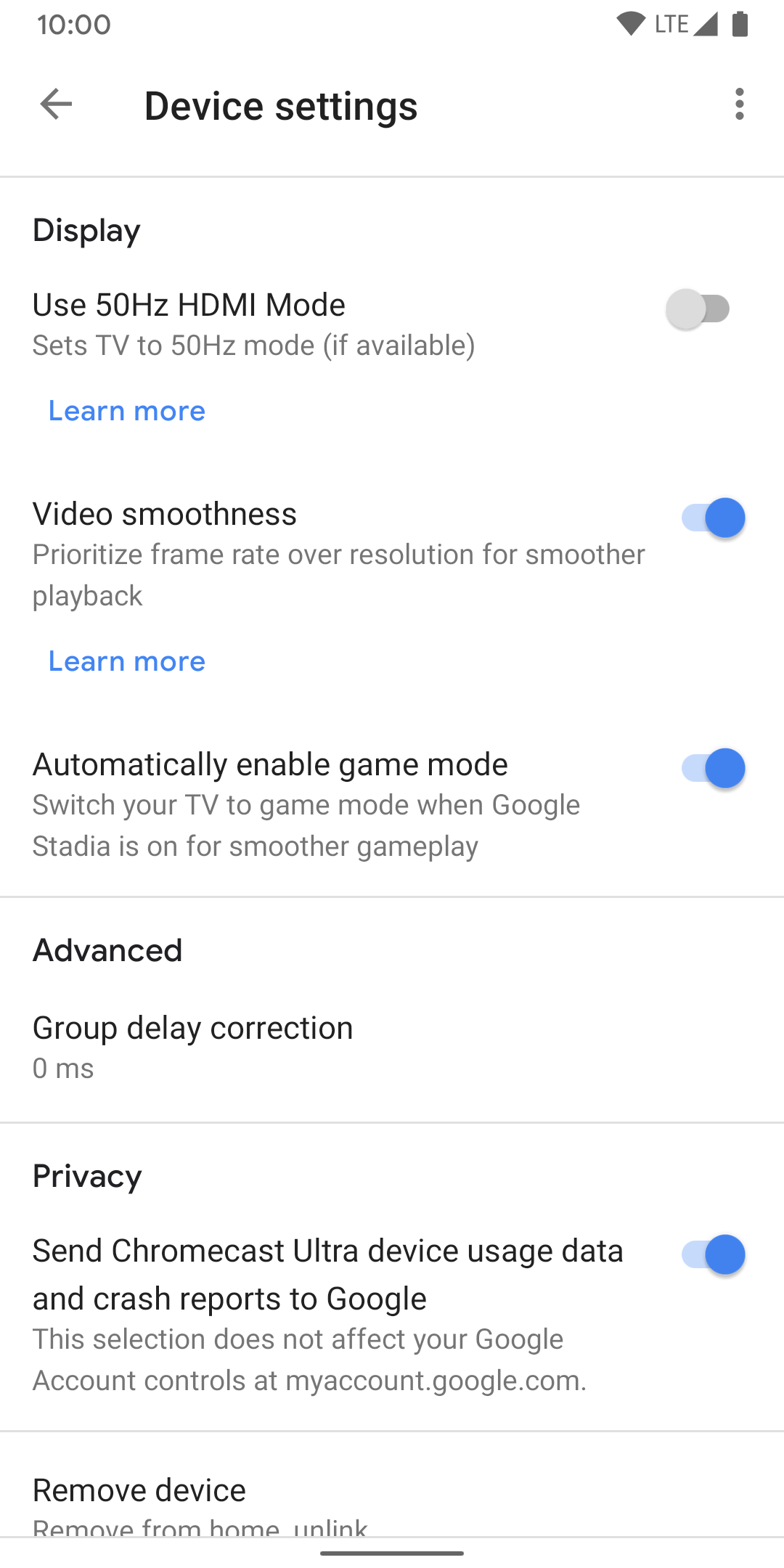A screenshot of the Android device settings page is displayed. The status bar at the top shows a 10:00 AM timestamp, Wi-Fi signal icon, "LTE" network status with full bars, and a fully charged battery icon. Under the header "Device Settings," a back button and a vertical three-dot menu icon can be seen. The first option reads, "Display: Use 50 Hz HDMI mode to set the TV to 50 Hz mode if available," accompanied by a gray toggle switch indicating it is turned off. Below, the "Video Smoothness" setting is enabled with a blue toggle switch. It prioritizes frame rate over resolution for smoother playback, with an option to "Learn more." Next, the "Automatically Enable Game Mode" option is also switched on with a blue slider, which activates game mode for smoother gameplay when Google Stadia is in use. Under the "Advanced" section, "Group Delay Correction" is set to zero microseconds. In the "Privacy" section, the setting to "Send Chromecast Ultra device usage data and crash reports to Google" is enabled, indicated by a blue slider. A note clarifies that this selection does not affect Google account controls at myaccount.google.com. Finally, at the bottom, options to "Remove Device," "Remove from home," or "Unlink" are provided.